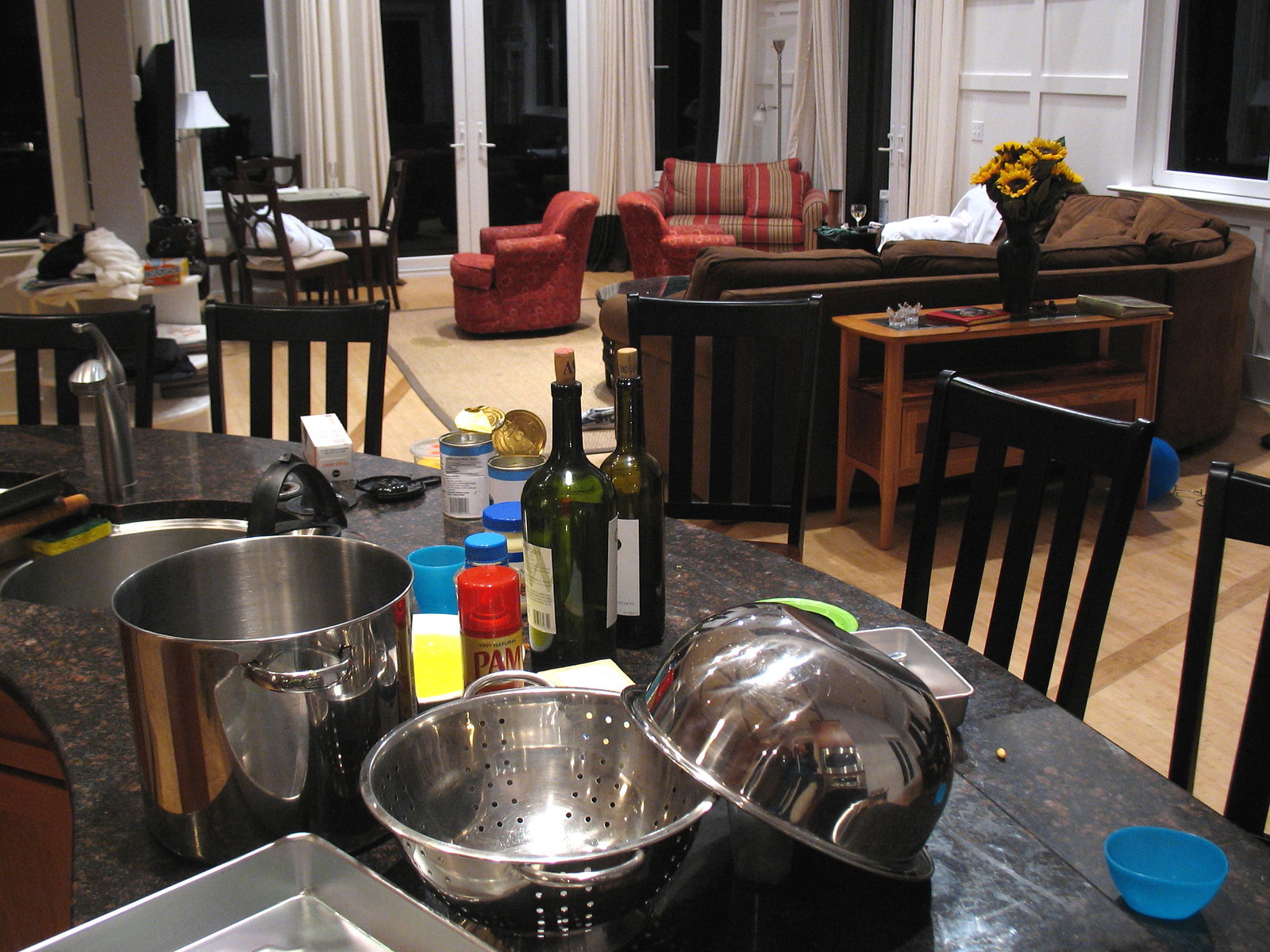In this image, the foreground features a visually intriguing living room setup. On the left side, there's a stylish table with a unique black and brown granite marble tabletop, boasting a slightly curved shape. Positioned near the bottom of the image, you notice a large, several-gallon silver pot accompanied by a big silver strainer with holes. A smaller silver bowl, seemingly designed to fit atop the pot, is placed off-center. 

Nearby, a sleek silver tray holds two wine bottles, which are greenish-brown in color and sealed with corks. Among other items on the table are a red container of Pam grease spray, various white containers with blue lids, and open cans with gold tops. A plastic blue cup adds a pop of color, and a small circular sink is visible, complete with a green sponge beside it.

Surrounding this table are five wooden chairs characterized by their high backrests with vertically aligned wooden planks. In the background, the living room area is furnished with a large brown sectional couch, positioned in front of a brown wooden cabinet featuring a vase filled with vibrant sunflowers. Meanwhile, a cozy red two-seater sofa, adorned with tan stripes, sits across from the sectional, accompanied by a matching one-seater red sofa. 

The living space is unified by a tan beige area rug and illuminated by windows draped with long, floor-to-ceiling white curtains that are drawn to the side. Revealed beyond the curtains is a dark, night-time scene, hinting at a possible patio door adjacent to the windows. The entire setting exudes a warm, homely ambiance perfect for relaxation and social gatherings.